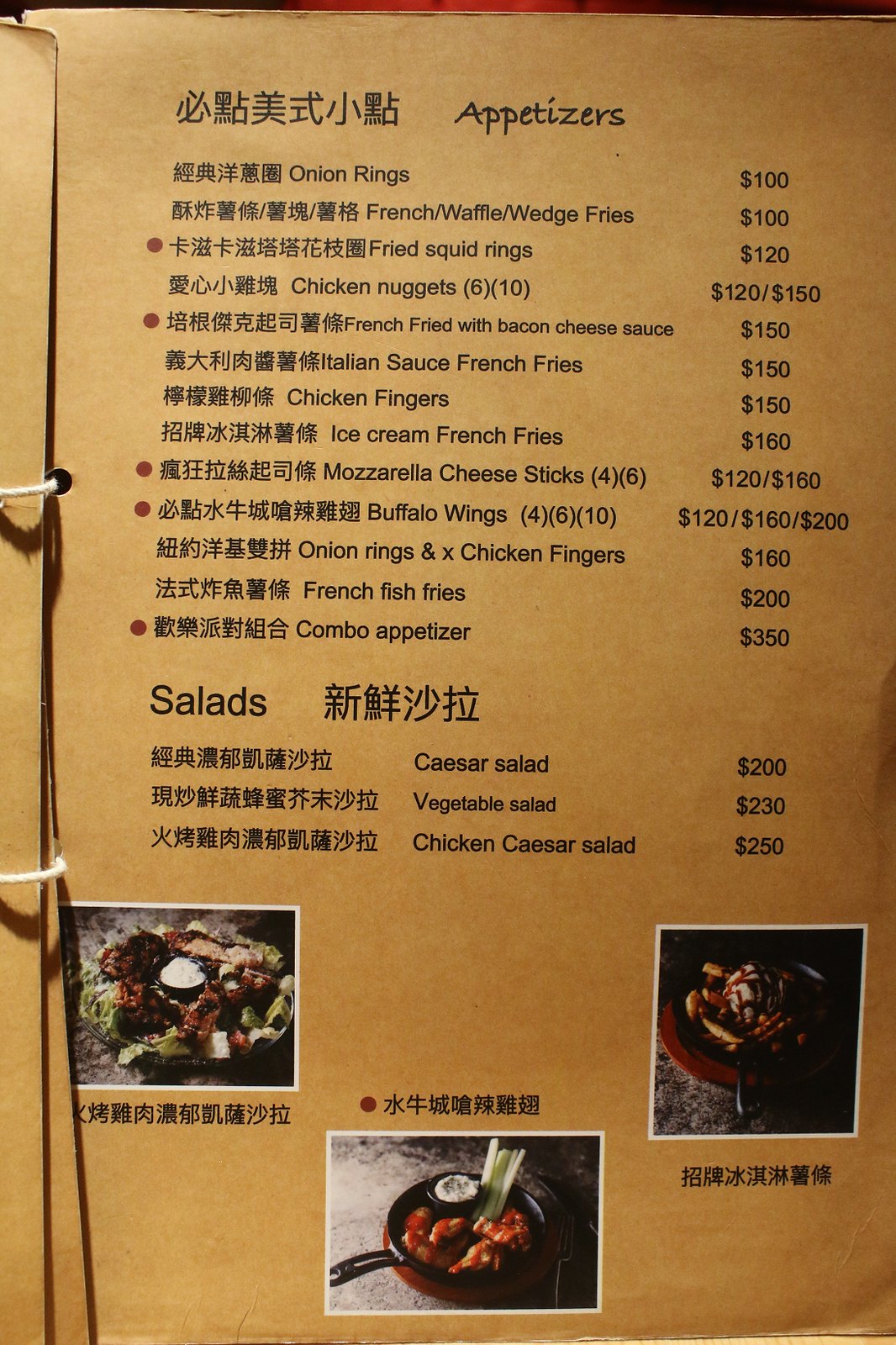In this color photograph, presented in portrait format, we see the right-hand page of a multi-page menu from a Japanese or Chinese restaurant. The menu, which overall appears to consist of at least three pages, is kept together by a white string threaded through punched holes, with the first two pages flipped to the left. 

The background of the page is a light brownish hue, providing a warm, inviting contrast to the black text displayed upon it. Towards the bottom of the page, three vivid images showcase different food dishes, though the captions accompanying these images are written exclusively in Chinese or Japanese, making it difficult to identify the specific meals.

At the top of the page, the textual content is organized into two sections: "Appetizers" and "Salads." Under the appetizers heading, a variety of options are listed with their prices: Onion Rings for 100 (currency unspecified), French Waffle Wedge Fries for 100, and Fried Squid Rings for 120, among others. Following this, the salads section offers a Caesar Salad for 200 and a Vegetable Salad for 230. The high numerical values imply that the currency used is likely not familiar to Western standards, suggesting a price system unique to the local economy.

Overall, the menu's design and pricing evoke curiosity and cultural intrigue, with the tantalizing images hinting at the gastronomic delights that await patrons.